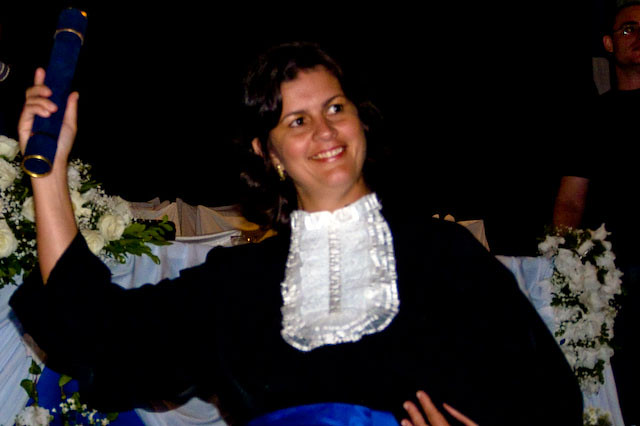This photographic image captures a white woman in her thirties or forties, standing indoors against a very dark background, prominently illuminated. She has long, curly black hair and wears a long-sleeve black shirt adorned with a white, elaborate lace front piece resembling a bib. Her ears are decorated with gold ring earrings, and a green belt cinches her outfit around the waist. The woman is holding up a microphone with her left hand, while her right hand rests on her hip. She appears to be at some form of cultural or ceremonial event, smiling warmly. The background features a table draped in a white tablecloth, flanked by bouquets of white roses. Alongside, a man in a black t-shirt and glasses is faintly visible. The overall atmosphere hints at a celebratory or special occasion, possibly highlighting the woman's central role in the event.